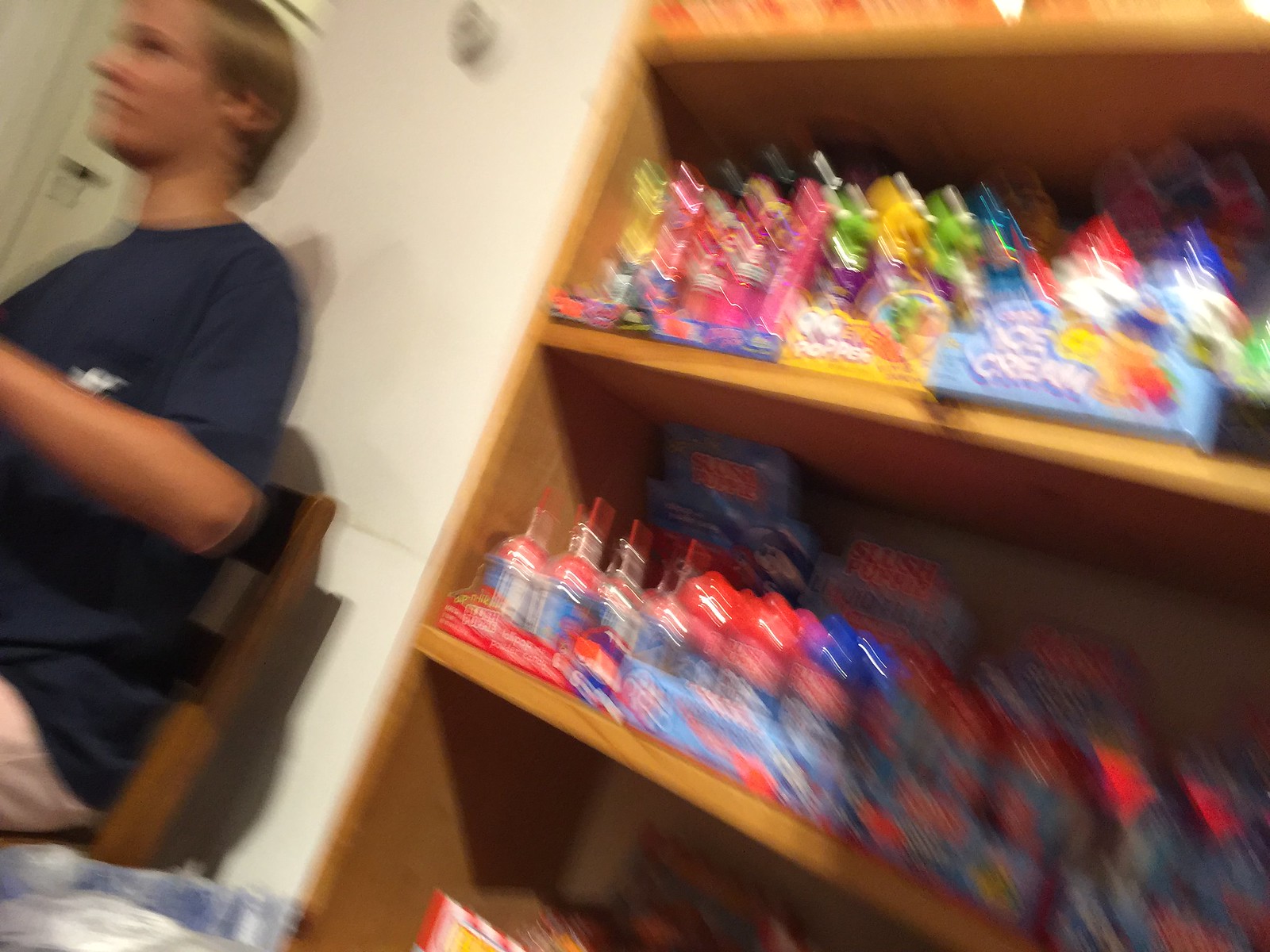This photograph captures a young Caucasian individual, between 20 and 30 years old, with a light skin complexion and medium-length blonde hair, seated in a simple wooden chair. The person is wearing a navy blue t-shirt with a white logo on the left side near the breast area and either black or white shorts or pants. The individual is positioned in front of a tall, light brown shelving unit, leaning slightly at an angle, making the details of the shelving contents hard to discern due to the photograph's blurriness. The shelves hold a variety of colorful candies, some in containers with blue packaging that are arranged in sets of six. These candies include pink, orange with green, light blue items, and bottle-shaped ones with red and blue details. Some candies feature ice cream-related themes and labels, with a notable occurrence of the "Slush Puppy" logo. The exact types and brands of candy are largely indistinguishable due to the image's poor quality. The scene is set against white walls, and there is a basic black bookcase visible from the right-hand side of the frame.